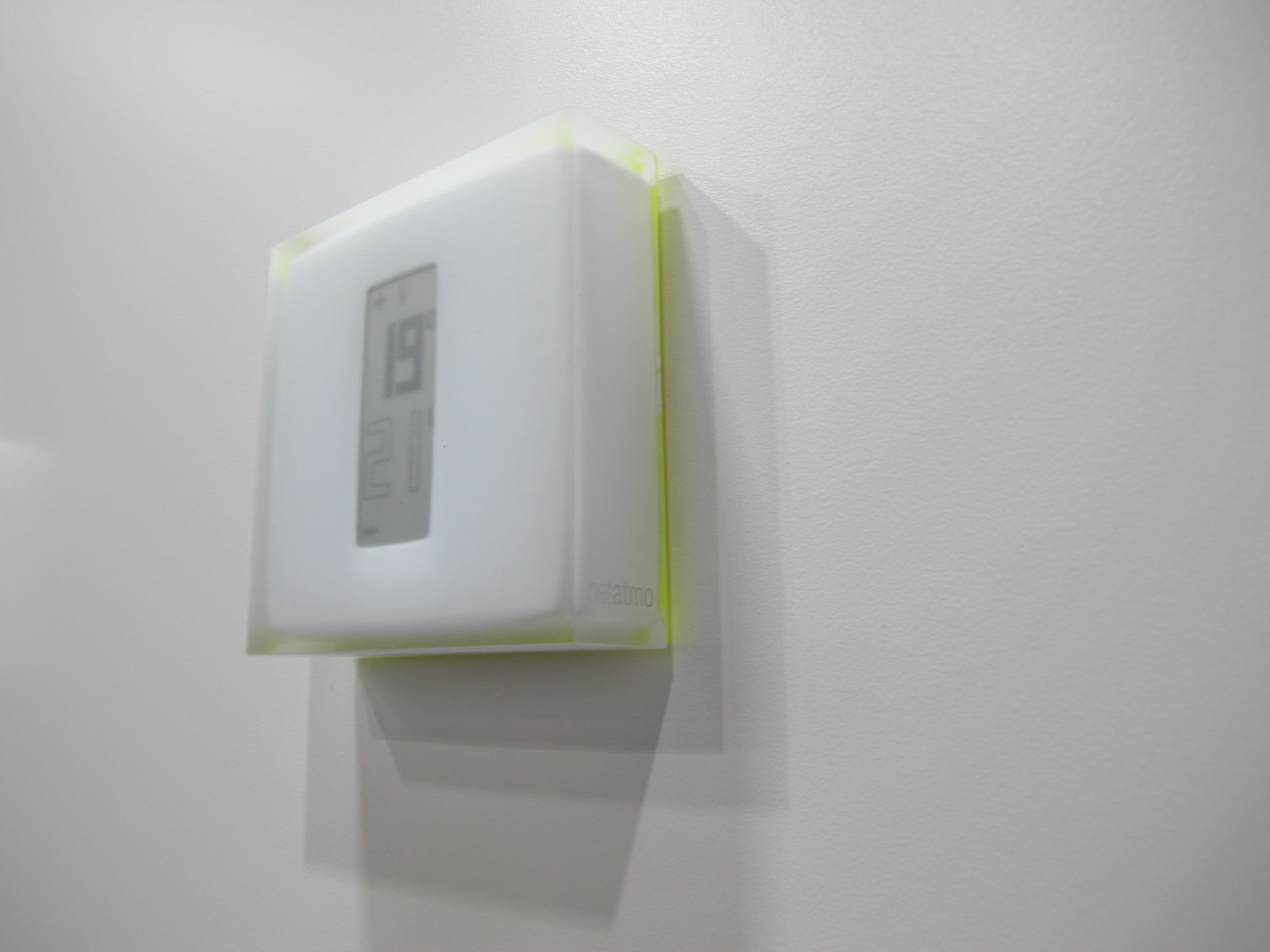This photograph is taken in landscape mode, capturing a thermostat mounted on a light gray wall. The thermostat is enclosed within a transparent protective plastic cover, designed to restrict unauthorized access to temperature adjustments. The protective cover has noticeable yellow edges, either due to a reflection or its actual color.

Positioned slightly towards the left side of the image, the thermostat's digital display is partly visible. The bottom right corner of the device bears a partially visible label, possibly reading "R-E-T-A-T-M-O." The screen features a plus sign (➕) at the top, followed by the number 19 in bold, dark digits, indicating the current set temperature. Below the 19, the number 21 is displayed in lighter digits, suggesting the actual room temperature. A minus sign (➖) is also present, likely allowing for adjustments. The thermostat allows users to increase the set temperature using the plus sign to make the room warmer.